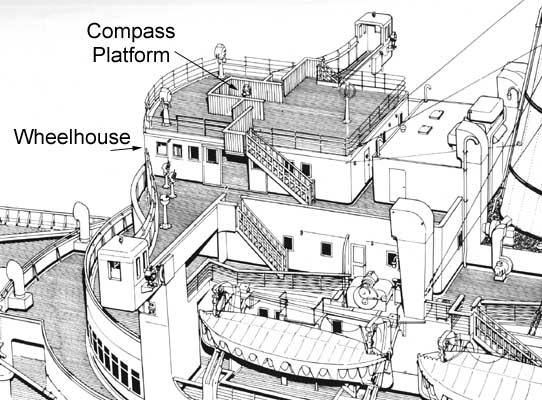The image is a detailed black-and-white line drawing, likely created using computer-aided design or pencil with bluish ink, depicting the top portion of a large ship with three distinct levels. At the very top is the "Compass Platform," explicitly labeled with text and an arrow pointing to it. Below the Compass Platform is the "Wheelhouse," also labeled with an arrow, which presumably is where the captain operates the vessel. Adjacent to the Wheelhouse is an outlook area equipped with viewfinders for observing the ocean. The third level down houses additional emergency boats or lifeboats, two of which are visible in the drawing. The ship’s structure is interconnected with various wires, cranks, and stairs that lead between the levels, enhancing the complexity and functionality of the vessel. The overall setting of the illustration is clean, with the background remaining plain white.